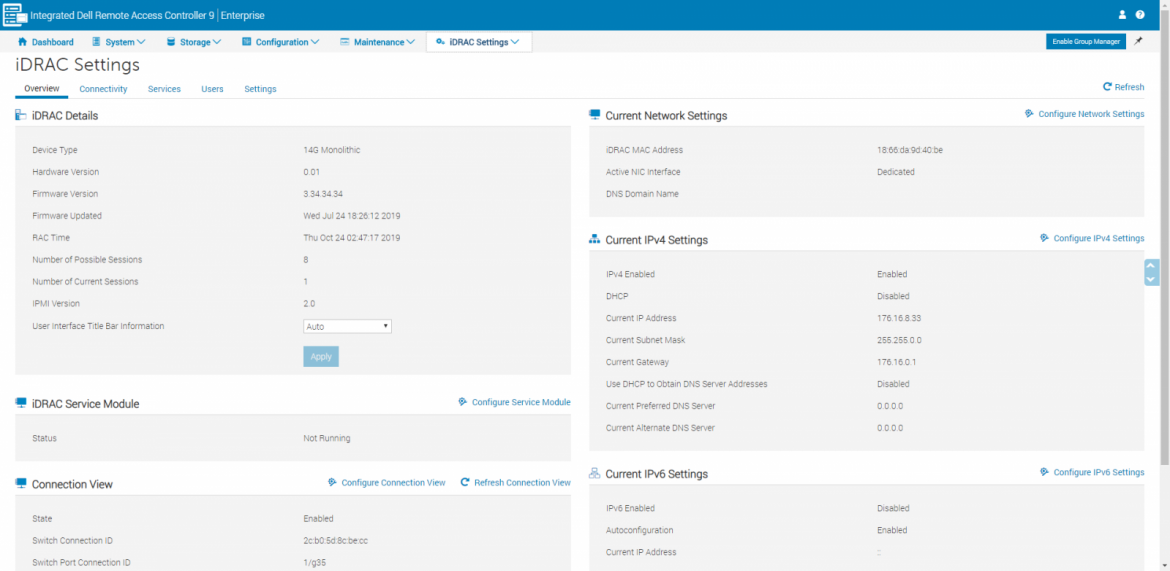A detailed screenshot of a network settings software interface is displayed against a clean white background. The interface features several light gray rectangles organized into two columns. At the top of the page, a prominent blue bar contains white text that reads "Integrated Dell Remote Access Controller 9 Enterprise." In the upper right-hand corner of this bar, there is a sign-in icon. 

Below the blue bar is a thin gray navigation bar with menu options labeled: Dashboard, System, Storage, Configuration, Maintenance, and IDRAC Settings. Another menu bar beneath this is segmented into tabs that read: Overview, Connectivity, Services, Users, and Settings.

Occupying most of the page are the two columns, each containing three light gray rectangles. Each rectangle is outlined and contains varied numbers and text, presenting different headings in bold black font. This structured layout provides a comprehensive view of the network settings available within the Dell Remote Access Controller interface.